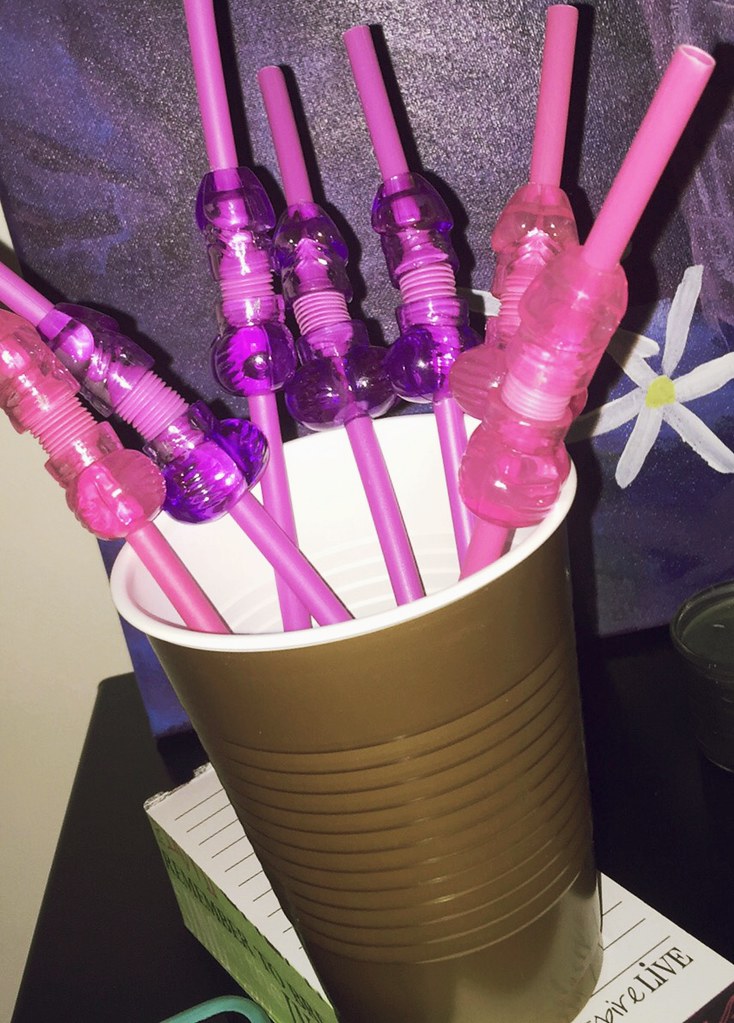The image features an extreme close-up of a smooth, flat, dark brown end table, likely in a home setting, possibly a bedroom or living room. On the tabletop rests a gold plastic solo cup with a white interior, which contains seven novelty straws—some pink, some purple—each adorned with a phallic shape near the top, extending past the middle but still offering ample straw length. The cup is positioned atop an index card or a notepad with green-edged paper, partially revealing the word "live." Behind this setup is a propped-up painting on canvas displaying an abstract blend of dark colors—purple, blue, and black—accentuated by a simple white daisy-like flower with a yellow center. A white wall serves as the backdrop for the vivid scene.